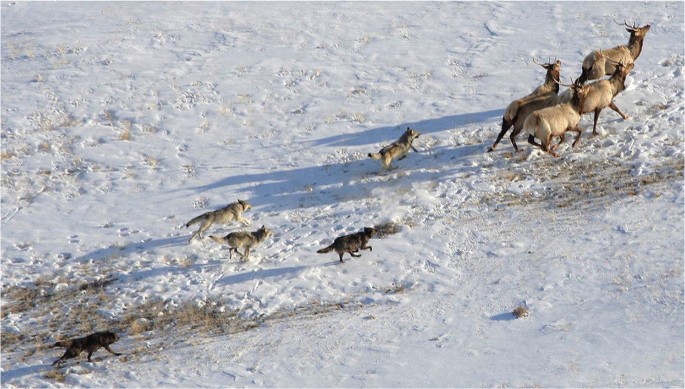In this overhead photograph, likely taken by a drone, we see a dynamic chase scene unfolding on a snowy terrain. The image captures five wolves in pursuit of four deer across an icy, snow-covered field. The deer, all light brown in color and adorned with large antlers, are grouped closely together in the upper right corner of the image, running at full speed with their heads held high. Their antlers vary in size, with the front deer sporting the largest set. Chasing them are five wolves, moving rapidly, their dark and light gray or brown fur stark against the white snow. Two of the wolves are black, with one prominently positioned in the lower left-hand corner of the image. The other three wolves have gray and white fur, with the lightest wolf trailing closest to the deer. The snowy ground beneath them is littered with footprints—hoof and paw prints alike—highlighting the frantic pace of the chase. Scattered vegetation and patches of exposed brown ground break up the expanse of snow, adding texture to the scene. The shadows of the running animals cast upon the snow enhance the sense of movement and urgency in this captivating wildlife moment.